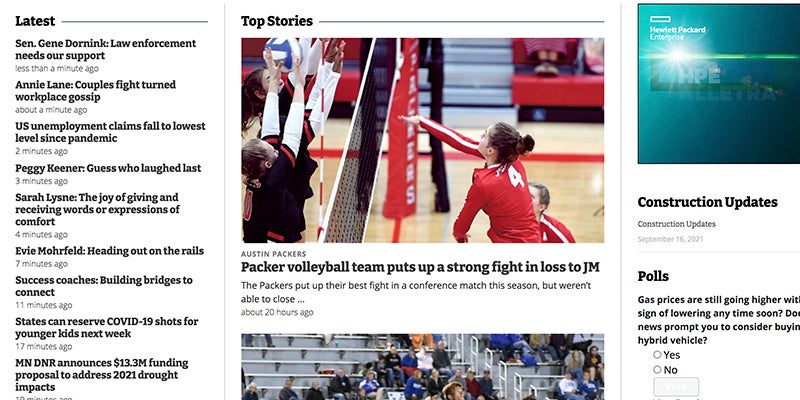This screenshot captures a local news website, offering a glimpse into the latest updates and key stories. The layout features a clean, white background that frames the content effectively. In the top left corner, the section labeled "Latest" is highlighted in black text. Within this section, nine clickable headlines provide a variety of news articles for readers, such as "US Unemployment Claims Fall to Lowest Level Since Pandemic" and "Success Coaches: Building Bridges to Connect."

Dominating the center of the image is a feature column titled "Top Stories," prominently displaying an action shot from a women's volleyball match. The photograph showcases players in red and black uniforms mid-game. Beneath this dynamic image, the headline reads, "Packer Volleyball Team Puts Up a Strong Fight and Lost to JM," likely recounting the latest high school or local college volleyball match.

Positioned at the top right is a teal advertisement box for Hewlett Packard Enterprise, adding a splash of color and commercial content to the page. Below this ad, in the bottom right section, are additional hyperlinks directing readers to updates on local construction and a poll concerning gas prices in the area.